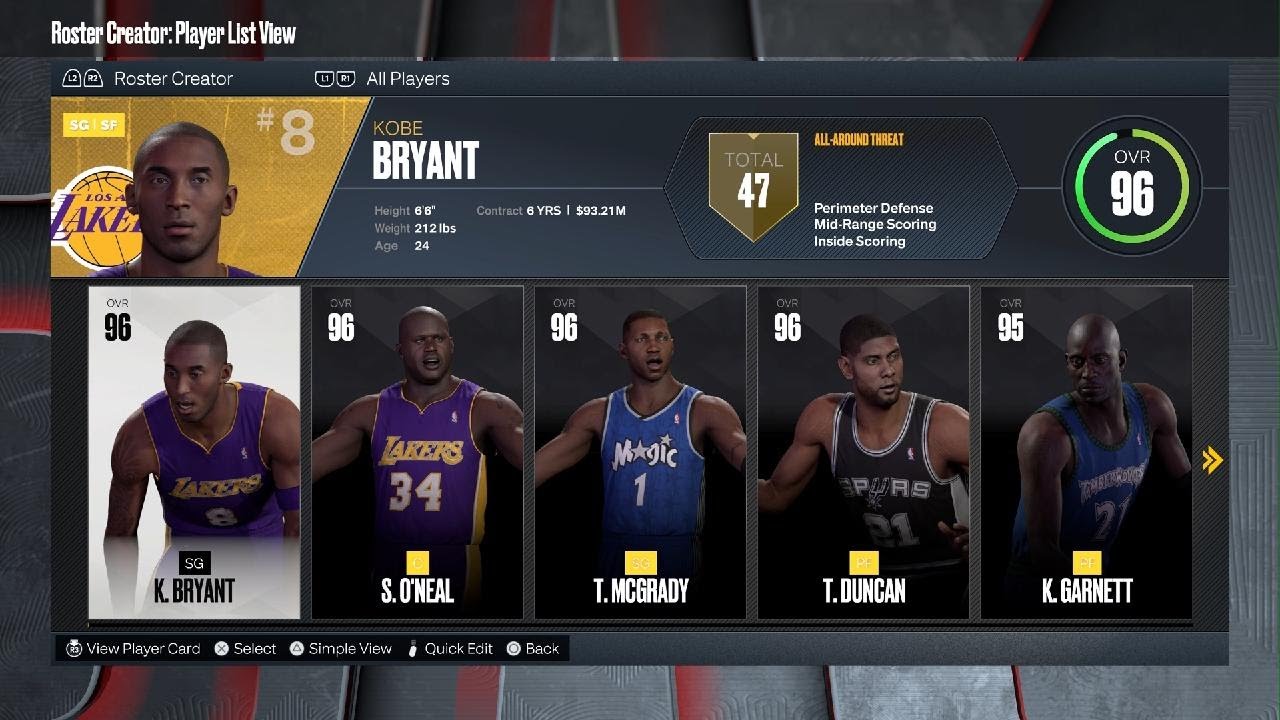A detailed player profile page in a video game is depicted. At the top left, the header reads "ROSTER CREATOR: PLAYER LIST VIEW" in a bold white Impact-style font. Below this header, there is a rectangular section with a dark blue background designed to appear slightly three-dimensional towards the left. 

In this rectangular section, a Lakers player with short black hair and a five o'clock shadow is prominently featured. Positioned to the back left of the player is a basketball and the Lakers logo. At the top right corner of this area, the number "8" is displayed in a semi-transparent white font.

To the right of the player image, in all-capital yellow lettering, "KOBE" is displayed lightly, followed by "BRYANT" in a bold white Impact-style font. Below his name, the player's stats are listed with the categories in light gray and the corresponding data in small, bold white letters. The stats begin with "HEIGHT: 6'8"" (possibly "6'6""), "WEIGHT: 212 LBS," and "AGE: 24." The contract details are listed as "CONTRACT: 6 YRS" with a small white line divider, followed by "SALARY: $93.21M."

Adjacent to this section is a small badge or trophy icon in a diamond shape that transitions into a square. It has "TOTAL: 47" written in a light gold font. To the right, in orange text, the designation "ALL-AROUND THREAT" is given.

At the bottom of the section, in white text, the player's key attributes are highlighted as "PERIMETER DEFENSE," "MID-RANGE SCORING," and "INSIDE SCORING."